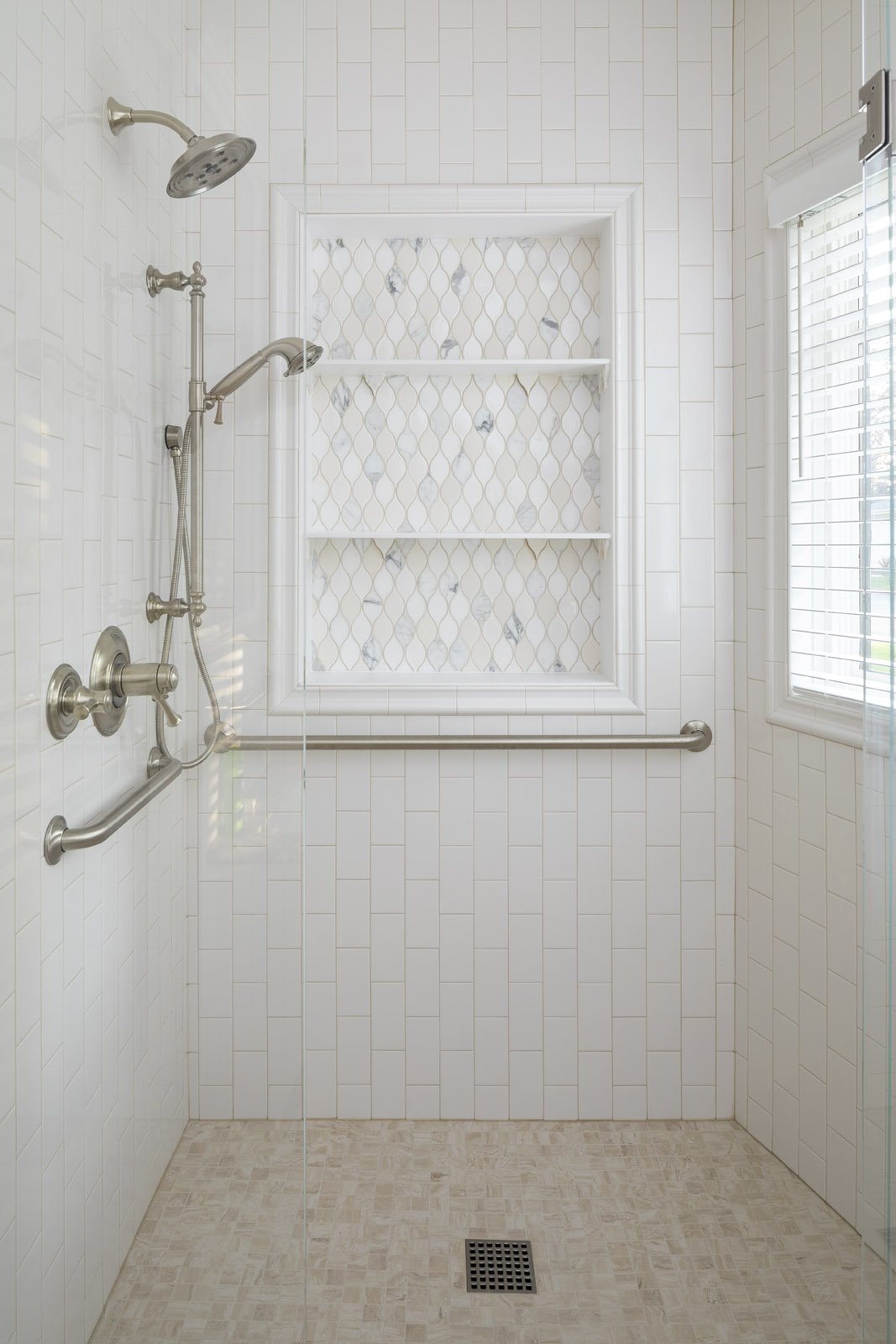The image depicts a spacious, modern shower with distinctive features. The shower area is tiled with light beige and white marble tiles, and the floor is composed of the same light beige marble with a central dark gray, square-shaped drain. There are two windows; one on the right wall, covered with Venetian blinds, and another in the background with a metal safety railing beneath it. The shower is equipped with both a fixed silver metal shower head on the wall and a handheld shower head for flexibility. Additionally, silver metal handlebars for safety are located on the left side and towards the back of the shower. The white wall features a tiled shelf with diamond-shaped patterns, adding to the decorative aspects of the shower space. Overall, the area exudes a clean and elegant aesthetic with a spacious feel.